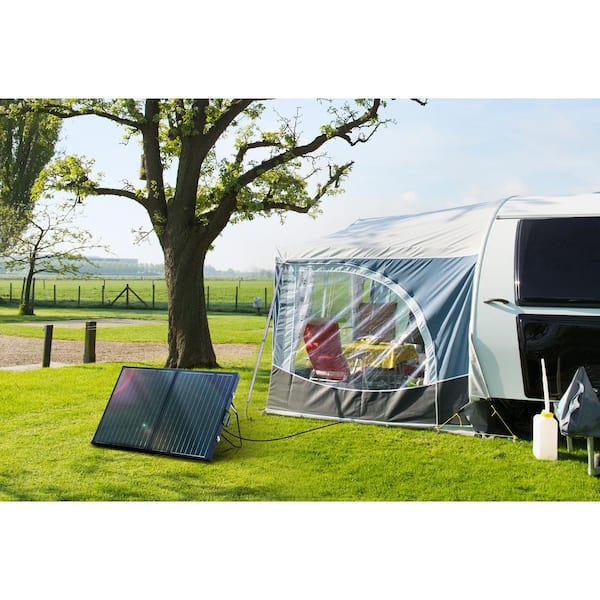In this outdoor image, set against a backdrop of lush green grass and a vibrant blue sky dotted with clouds, a cozy camping setup is depicted. The setup features a dual-structure arrangement, with a permanent, hard-shell camper painted in white and black alongside an attached blue-and-white tent. The tent is screened with clear netting and includes a zippered entrance. Inside, the tent contains red lawn chairs and a table adorned with a yellow tablecloth, creating a comfortable dining area protected from bugs.

A prominent solar array is visible outside, with wires extending into the tent area, ensuring a sustainable electricity source. The entire arrangement is situated under the shade of a large, leafy tree. To the right of the tent, a jug with a spout, white with a yellow top, is clearly seen. In the distance, there is a picturesque view of a green field bordered by a pasture and small trees, enclosed by a distant fence. This idyllic scene captures a blend of nature and modern camping conveniences.